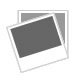This image is a cropped, mostly square photograph taken indoors, measuring approximately three inches by three inches. The background is a white sheet with visible rolls and folds, indicating it hasn't been perfectly flattened. At the center of this photograph is a handmade wool garment, potentially a cloak, cape, or poncho, which is buttoned down the front and features slits on either side for the arms.

The garment has a distinctive red folded collar. The shoulder area starts with bands of red and white stripes, followed by gold, black, and another gold band. The midsection, which covers the torso, is a light cream color and adorned with vertical red geometric designs on either side of the buttons, resembling diamond shapes within rectangles. 

Towards the bottom, the pattern repeats the initial sequence: gold, a thick black band, another gold band, followed by red and white stripes. The garment ends with a thick red band at the very bottom. Overall, the piece has a broad, slightly triangular shape, wider at the bottom, and is meticulously laid out on the white sheet.